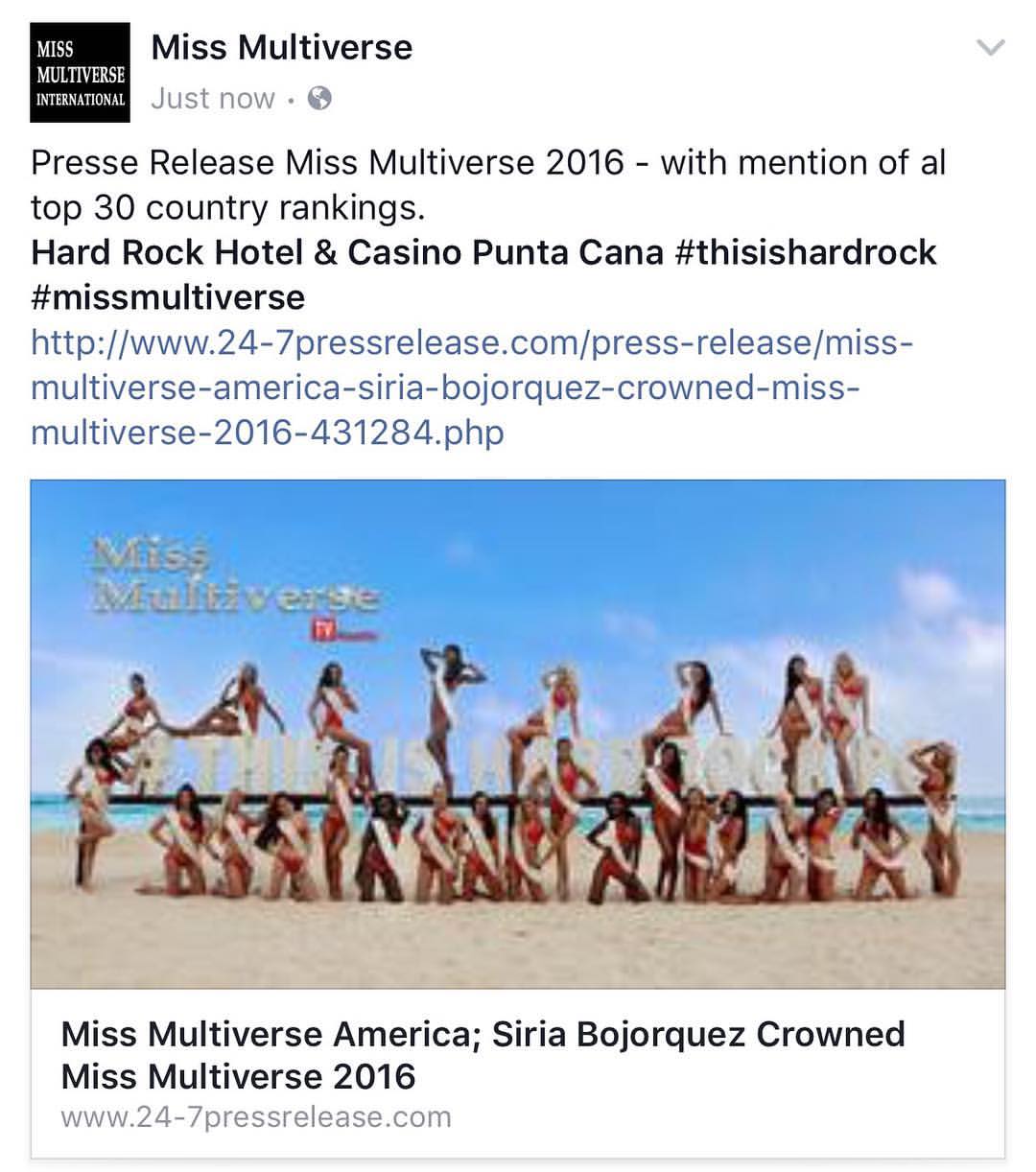A vibrant press release image captures an Instagram post from the Miss Multiverse International beauty contest. The photo, set on a picturesque sandy beach with calm waters and a clear blue sky, showcases the contestants of Miss Multiverse 2016. About 30 to 35 women, all dressed in matching red bikinis and white sashes, pose confidently. Some kneel in the foreground sand, while others stand above them, creating a dynamic composition. The image features the Miss Multiverse logo and the title prominently in white letters. Text details include rankings for the top 30 countries, and the venue, Hard Rock Hotel and Casino Punta Cana. At the bottom, it proudly announces Miss Multiverse America, Serreria Bojorquez, crowned Miss Multiverse 2016. The announcement provides links to the Miss Multiverse website, enhancing the excitement and accessibility of the event.